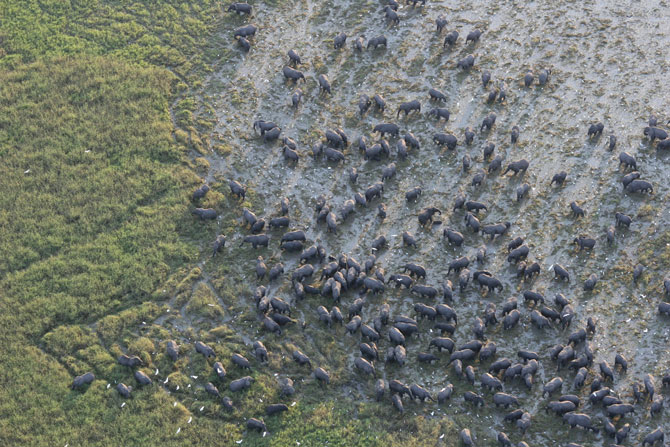This captivating aerial photograph captures an expansive herd of elephants in the wild, viewed from a high vantage point, possibly a drone or airplane. The elephants, large and small, are spread out across the landscape in a dense, uncountable throng, many of them appearing to be moving and foraging. The left side of the image is lush with green vegetation, including grass and bushes, indicating an area not yet heavily grazed. In stark contrast, the right side is mostly barren, with patches of greenery stripped away, revealing a white-silver colored ground beneath, likely due to the elephants' feeding habits. Amongst the elephants, several white birds can be seen flying, adding to the dynamic nature of the scene. This high-altitude shot emphasizes the scale and activity of the herd, set against the contrasting textures of verdant and depleted land.